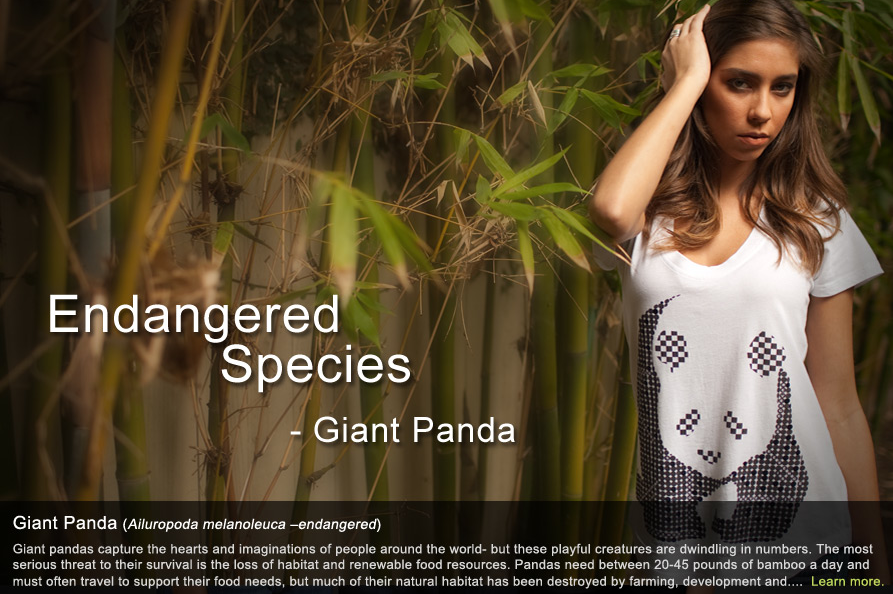This detailed photo advertisement features a young brunette woman standing among a dense backdrop of bamboo, with a slightly foggy ambiance. She has her right hand resting on her head and her neutral face slightly tilted to the right. The model is wearing a white t-shirt displaying an artistic, stitched-looking panda with black legs, ears, and nose against its white face. Prominently, in all capital white letters to the left of the woman, the text reads: "Endangered Species - Giant Panda." Below the photo lies a black background with further white text detailing the plight of the giant panda. It explains how these beloved creatures, faced with habitat destruction, require between 20 to 45 pounds of bamboo daily and often must travel to meet their dietary needs. The text emphasizes the critical threat of habitat loss due to farming and development. The caption on the black background concludes with the phrase "Learn more" in yellow, indicating further information is available, likely through a clickable link, reinforcing that this is an advertisement possibly for a conservation campaign or related merchandise.